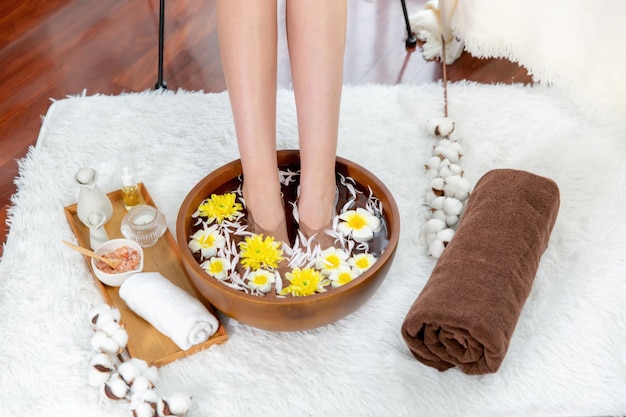This is a detailed color photograph depicting a serene indoor spa scene. Central to the image is a round wooden bowl filled with water, floating white flowers with yellow centers, and yellow flowers with green centers. A pair of woman's feet and legs, visible from the calves down, are soaking in the bowl. The scene is set upon a fluffy, white shag rug. To the right of the bowl lies a neatly rolled brown towel. To the left, there's a rectangular wooden tray holding various spa implements, including glass jars for scrubs, salts, and oils, a small candle, what appears to be a bottle of perfume, and a container with a wooden spoon. Sticks of cotton flank both sides of the bowl, enhancing the natural, relaxing ambiance. The backdrop features a polished dark brown wooden floor, and the legs of a black wrought iron chair from which the woman is seated are visible at the top of the photograph.